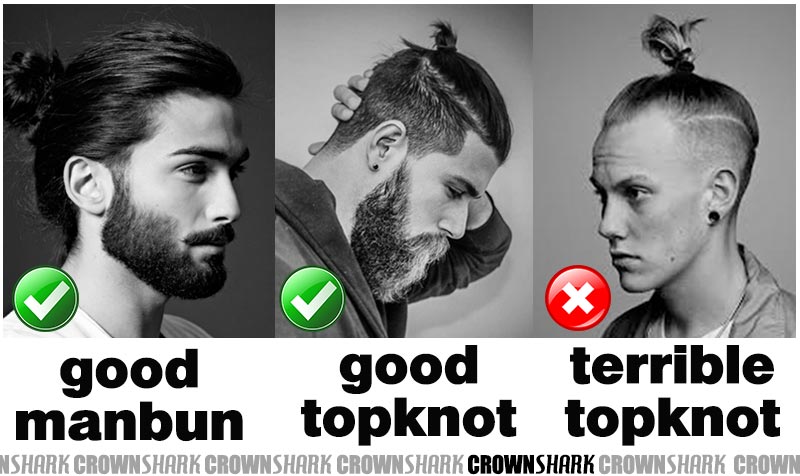This is a horizontally-oriented image divided into three vertical columns, each featuring a black-and-white photo of a different man with styled hair. 

In the first column, a man with black hair slicked back into a man bun is seen looking off to the right. He sports a goatee and a beard. Below his image, the text "Good man bun" is written in black letters, accompanied by a green circle with a white check mark in the bottom left corner.

The middle column displays a man with his head tilted downward. He has dark hair pulled into a top knot situated towards the back of his head and a longer beard. The text "Good top knot" is written below his image in black letters, also with a green circle and white check mark.

In the third column, another man, this one clean-shaven, is captured looking to the left. His dark hair is gathered into a prominent top knot on the crown of his head. Below his image, the text "Terrible top knot" appears in black letters, with a red circle and a white X in the bottom left corner.

Additionally, at the very bottom of the image, the words "crown shark" are repeated multiple times in gray text, interspersed with the same phrase in black text.